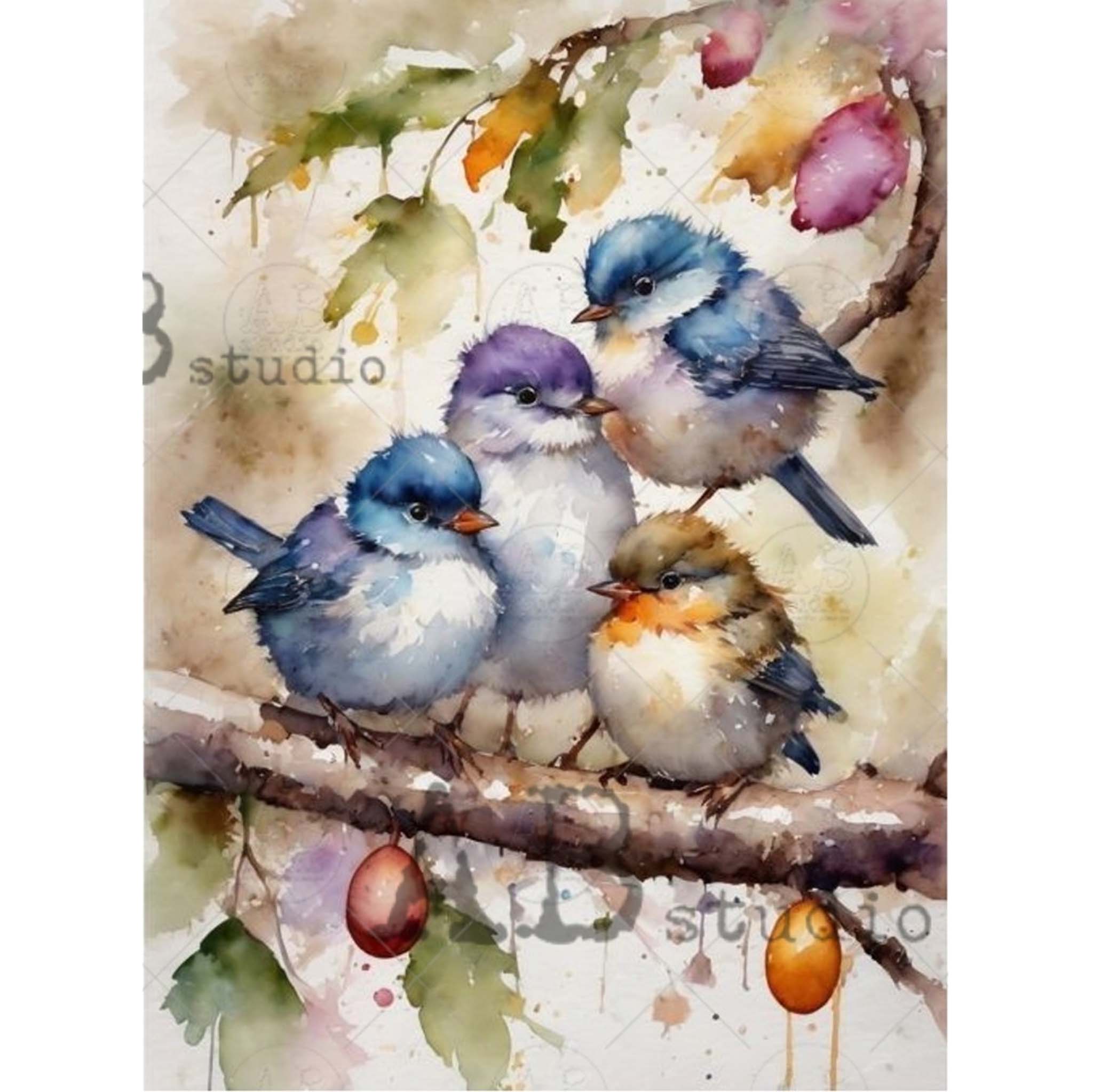This painting, executed in an impressionist or watercolor style, vividly depicts four small birds, potentially sparrows or parakeets, perched and fluttering on a tree branch. The scene is detailed with intricate colors and textures, focusing on the birds and their natural setting.

From left to right, the first bird stands out with blue feathers on its head, and white plumage on its underside, complemented by purplish-blue wings and tail feathers. It sports brown legs and black beady eyes. Above the branch, there's another bird appearing to flap its wings or alight, sharing similar blue hues.

The central bird is the largest, predominantly purple on its head and upper body, with a stark white underbelly. It has brown legs and a brownish beak, framed by the same striking black eyes.

The third bird, found to the right, showcases a blend of orange and brown on its head, with a white underside. Its wings and tail feathers are primarily blue, and it too has a brownish beak and legs.

The fourth bird, slightly overlapping with the branch above the main one, features a blue head and top section, white underbelly, yellowish beak, and bluish wings and tail feathers.

The tree branch supporting these birds is a mix of brown, white, and gray shades, with additional branches extending upwards. Decorating the branches are green and orange leaves, and clusters of round berries—red and orange—that bring a vibrant touch to the overall scene. Intermittent purple and pink flowers add to the natural beauty. 

Beneath the branch are egg-shaped objects, a pink one and an orange one, suggesting either artistic embellishments or symbolic elements. The painting is signed with "studio" in various places in shades of white, gray, and brown, contributing to its artistic charm.